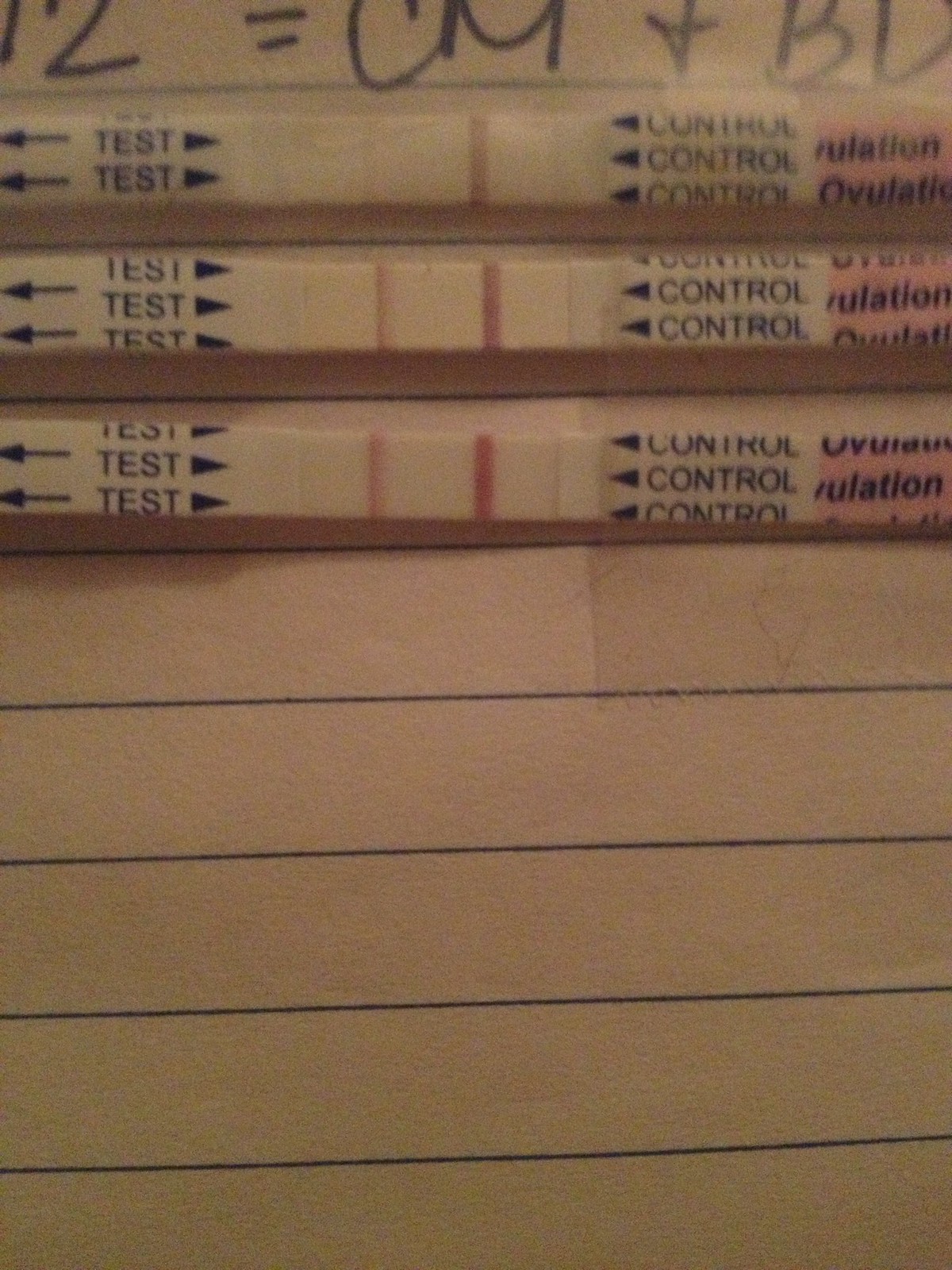A vertically oriented close-up image features three ovulation test strips, prominently showing the results area centered in the frame. The closely cropped composition reveals only the central test zones of the strips, each marked with distinct indicators. The image also includes a portion of handwritten text at the top, partially legible, reading "12 = cm + BL," written in black ink. The background is tinted in a brown or reddish hue due to indoor lighting conditions.

The test strips are aligned in stacked rows, positioned one above the other, leaving five blank rows below. The results on the test strips are highlighted by arrows pointing towards the "Control" area on the right, each displaying a dark reddish-brown line, and towards the "Test" areas on the left, which also feature pointed annotations.

This detailed presentation suggests the strips are related to ovulation tracking or potentially pregnancy testing, designed to provide vital reproductive health information.